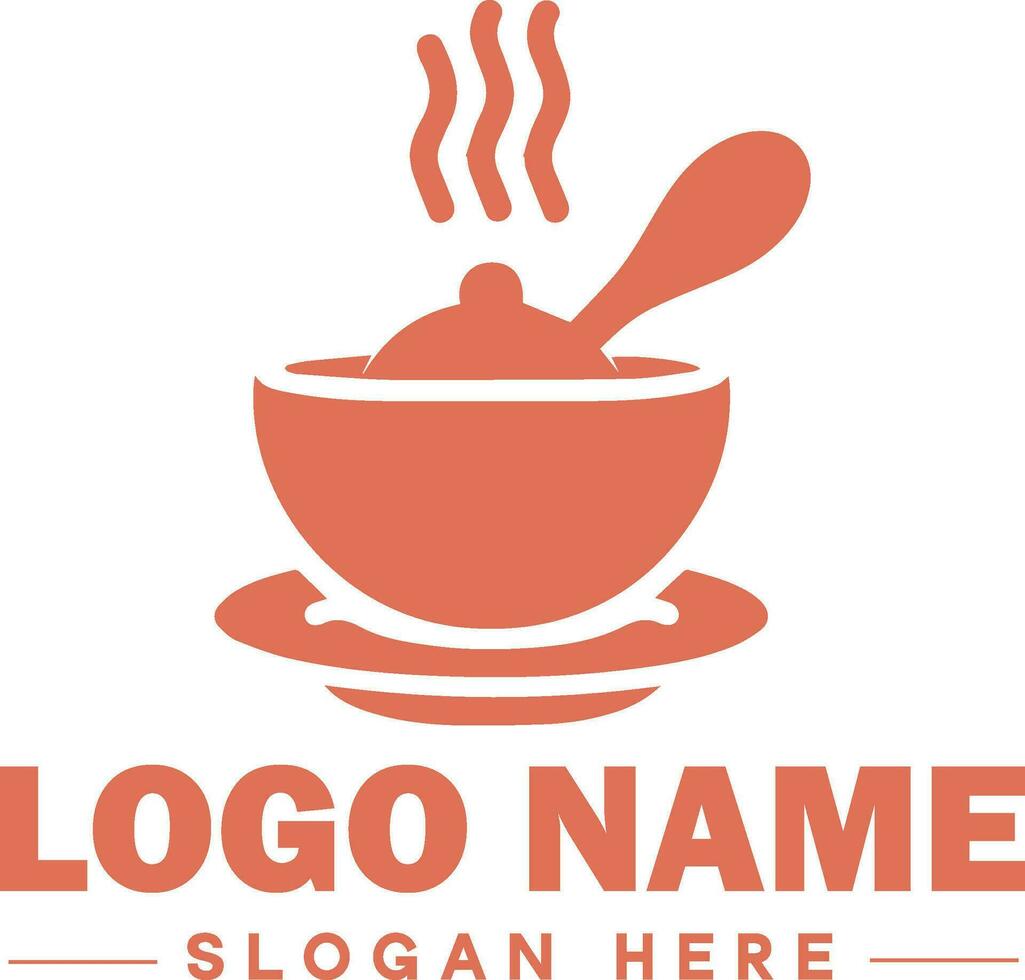This image features a logo on a plain white background. At the top center, there is a stylized silhouette of a bowl with a spoon, resting on a saucer. Above the bowl are three squiggly lines, representing rising heat or steam, indicating a hot food item. The entire icon, including the bowl, spoon, steam, and plate, is depicted in a dark pink color. Below the image, in the same dark pink color, are the words "LOGO NAME" in bold, capital letters, followed by "SLOGAN HERE" in smaller, thinner capital letters. The design appears intended for use as an advertisement.